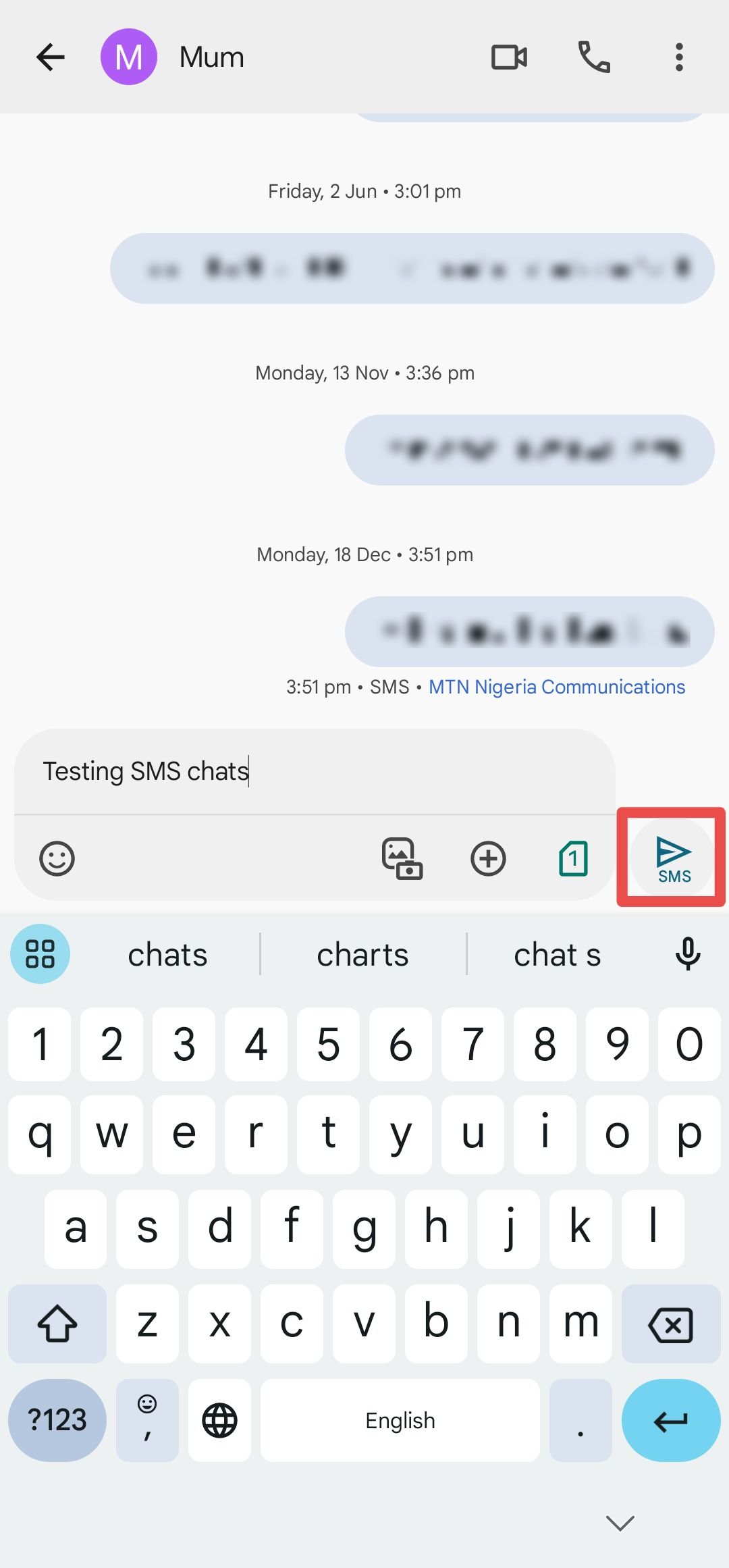A screenshot of a cell phone text message conversation. At the top of the screen, there is a gray header featuring a large, stylized "M" next to a purple circle. To the right of the circle, it says "MUM," indicating the contact's name. Positioned to the left of the purple circle is a gray arrow pointing to the left. On the right side of the header, there are three icons: a video camera, a phone headset, and an options menu.

The body of the text message display is light gray. At the top of this section, the date and time "Friday, June 2nd, 3:01 p.m." is centered and highlighted. Beneath this timestamp, there is an indication of a voice message, represented by a waveform image. This area might also represent edited or redacted messages, as it is blurred and appears with black boxes.

Following this, the text conversation continues with another timestamp marked "Monday, 13th of November at 3:36 p.m." and an additional one on "Monday, 18th of December at 3:51 p.m." Directly beneath the December timestamp, there's a line of text reading "3:51 p.m. SMS Mountain Nigeria Communications." Below that, in gray text, it says "testing SMS chats."

At the bottom of the screen, there is a red box covering the "send" button, which is situated to the right of a chat bar or text input box. The phone's keyboard is visible at the very bottom of the screenshot.